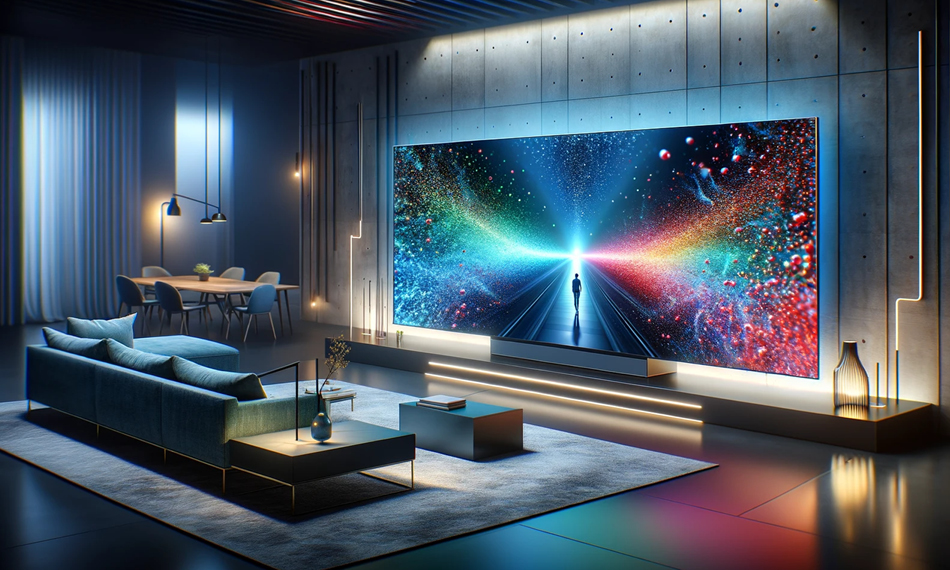The photo captures a contemporary, dimly lit room that combines a living and dining area with clean, modern aesthetics. In the living room, there's a spacious L-shaped teal sofa with a chaise lounge on the left, accompanied by a black side table holding a blue vase with a branch or plant. In front of the sofa is a black coffee table with a book resting atop it. Highlighting the media aspect of the room, a massive, home-theater-like TV screen dominates the right wall, which is covered with metal or concrete panels featuring rivets or small black dots. The TV screen itself shows a dramatic scene: a man walking along a bridge or runway towards a bright, shining light, surrounded by colorful splashes and lights in rainbow hues.

To the left of the TV is a rectangular light beige wood dining table surrounded by six gray chairs, arranged with two on either end and two on each long side. Above the table, pendant lights hang down, casting a soft glow over the setup. The dining area is backed by tall, white curtains, suggesting the presence of a window behind them. The floor features a gray rug that ties the entire space together, creating a cohesive and inviting atmosphere.